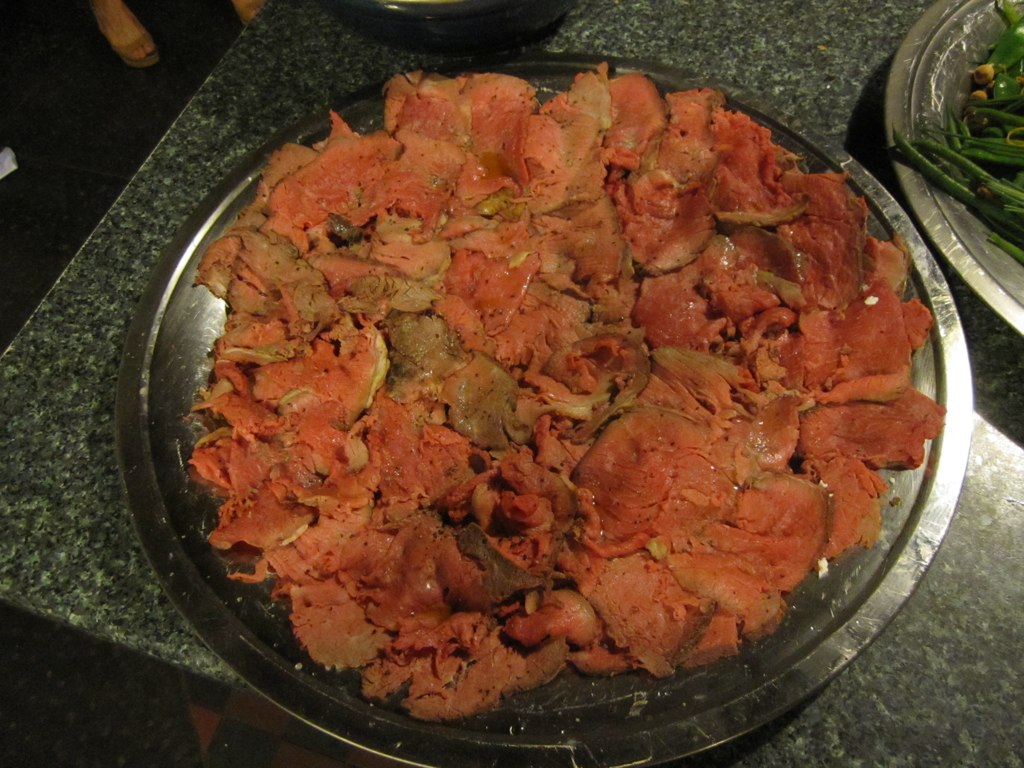This color photograph, taken indoors under somewhat dull artificial lighting, showcases a round silver platter meticulously arranged with thinly sliced roast beef. The pink and juicy meat slices are sprawled out flat, dominating the majority of the image's center. The platter rests on a speckled Formica or granite counter, contributing a grey, texturized backdrop to the scene. In the top right corner, another platter partially appears, heaped with stir-fried green beans and a few scattered yellow blobs. Above the main platter, an additional black bowl, lightly illuminated on its rim, peeks into the frame. In the top left corner of the image, a tiny glimpse of someone's foot in heels is visible, adding a human element to the shot. The photograph's perspective is an overhead close-up, aimed slightly at an angle, allowing the viewer to fully appreciate the artful presentation of the food.